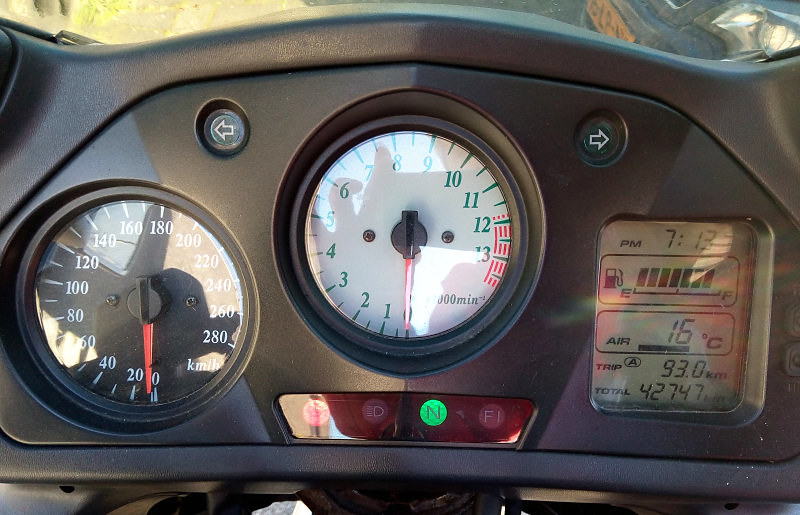This photograph showcases the intricate dashboard of a motorcycle or motorbike. Centrally positioned on the dash is a prominent white, round gauge likely serving as the tachometer, marked from 1 to 13. Adjacent to it on the left is a black speedometer ranging from 0 to 280. To the right of these gauges is a sleek square digital screen displaying various essential details: the time, noted as 7:13 p.m.; a nearly full gas meter missing just one bar; an air temperature reading of 16°C; Trip A distance of 93 kilometers; and an overall odometer reading of 42,747 kilometers.

The bottom center of the dashboard houses four indicator lights: a red light on the far left, a light symbol next to it, followed by a green "N" light, and an "F1" light. At the dash's top, flanking the central tachometer, are left and right arrow indicators, likely representing turn signals. The dashboard itself is a sleek black, and glimpses beyond it reveal a car in the top right corner and portions of a sidewalk, hinting at the vehicle's stationary position near a roadside.